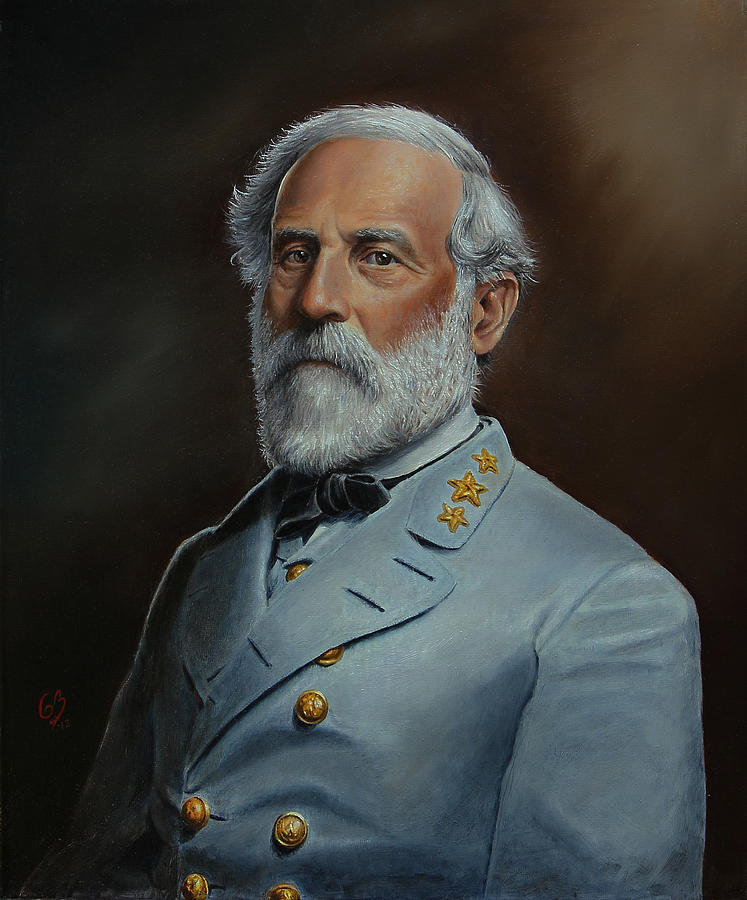This is a highly detailed, near-photorealistic portrait of Confederate General Robert E. Lee set against a rich brown background with lighter shading in the upper right-hand corner. Lee is depicted as an older man with white, slightly curled hair around his ears, a full, neatly trimmed gray beard and mustache, and dark brown eyes. His face shows a few wrinkles that add to his distinguished appearance. He is dressed in a light blue, almost powder blue, Confederate General’s uniform featuring a wide lapel with three gold buttonholes and two rows of three engraved gold buttons down the front. His uniform collar is adorned with three golden stars, which could either be embroidered or metal pins. Underneath his jacket, he wears a light blue shirt or vest with a gold button and a black cravat that resembles a bow tie. The portrait, signed with the initials 'GB,' captures Lee in a poised and dignified stance, with his body positioned in a three-quarter profile facing slightly to the left while he gazes directly at the viewer. The subtle play of light accentuates the details of his uniform and the texture of the background, enhancing the overall realism of the painting.